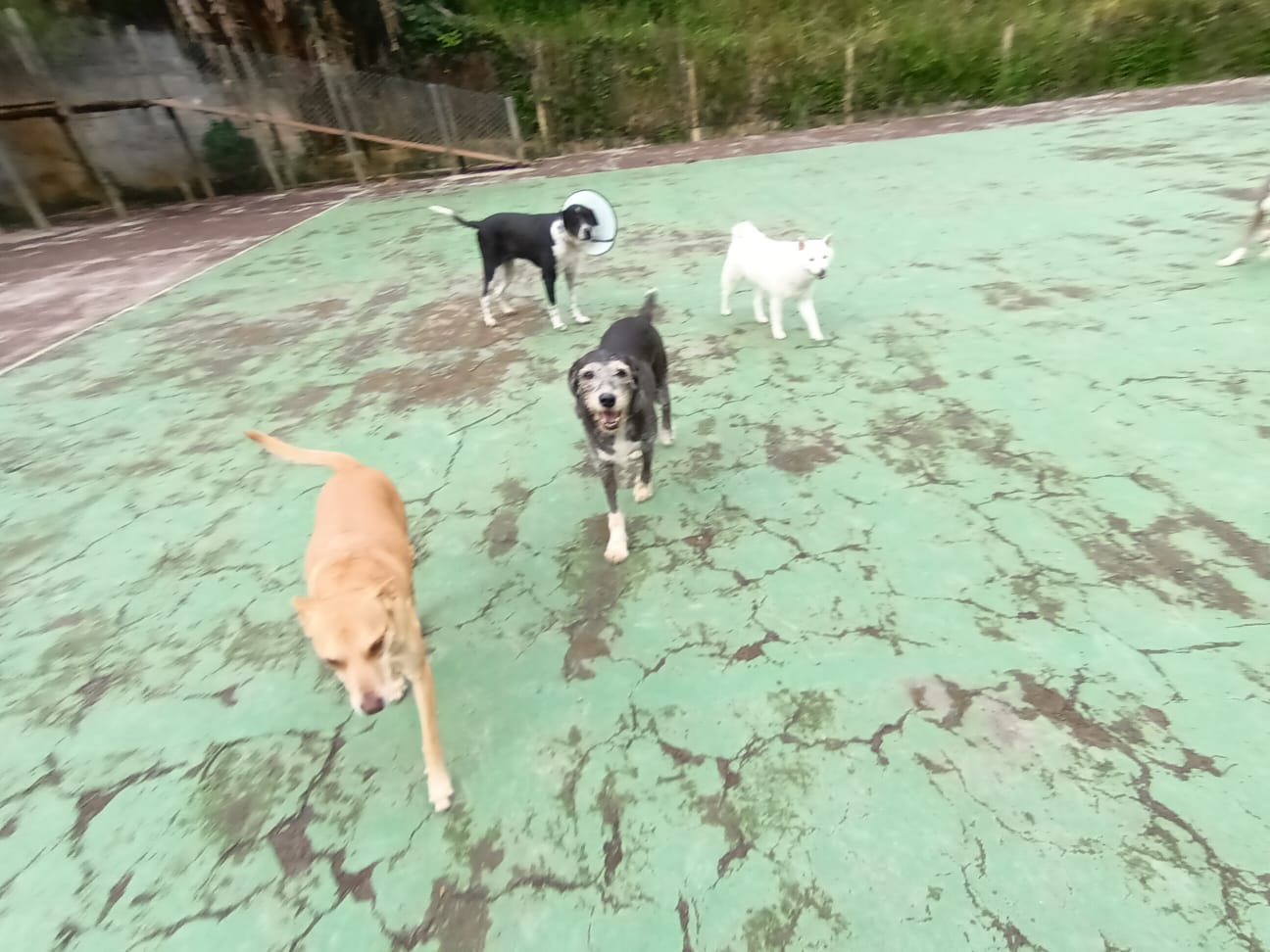The image captures an outdoor scene on an old, worn green concrete surface that might once have been a tennis court or similar recreational area. The floor is heavily cracked and the paint is faded, resembling a pistachio green color. In the foreground, there are five dogs: four fully visible and the partial legs and back end of another on the right side. The closest dog is all brown, while another is black with a white face and white paws. A fully white dog and a gray and white dog are also in the frame. The farthest dog, black with white on its chest, paws, and around its nose, is wearing a protective cone collar, suggesting it recently had surgery. The dogs appear to be moving towards the camera, giving the image a dynamic, slightly blurred look. In the background, there is vegetation including small trees and bushes, and a chain-link fence, possibly associated with a nearby stairwell or ramp leading to a different level. The setting feels like a neglected yard or sanctuary, perhaps in a warmer region like South America.